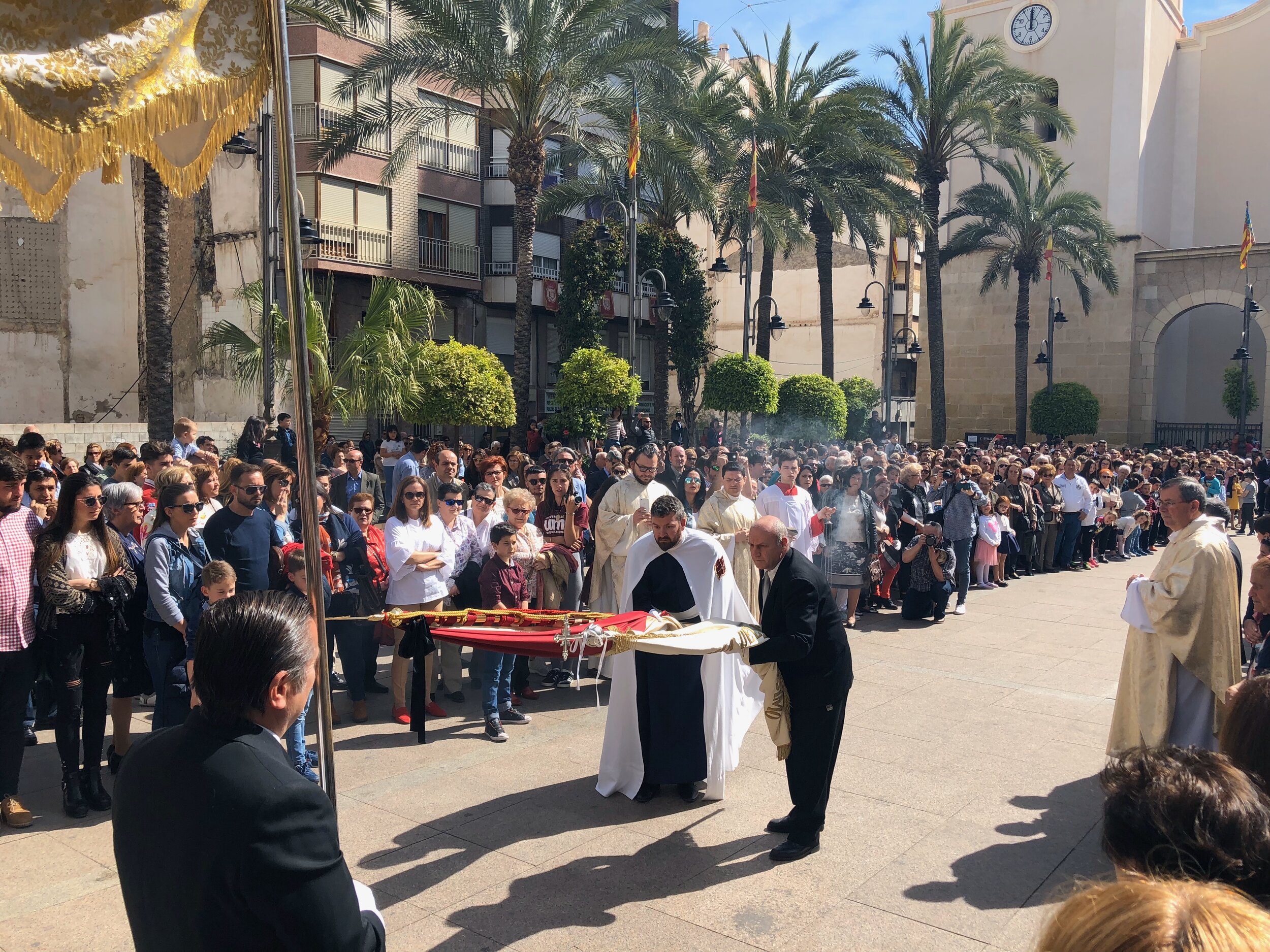In this outdoor image, a large procession likely related to a Catholic Church ceremony is taking place. The scene is set along a pathway lined with onlookers, most wearing sunglasses, under a clear, sunny sky. The crowd's attention is focused on two central figures: one bald man in a black suit, and another man with dark hair and a beard, dressed in black with a long white cape-like robe draping down to his feet. They appear to be holding a red and gold ornamental object, possibly a flag or ceremonial weapon.

To the left, another man in a black suit holds a pole topped by a springy canopy, while to the right stands another robed individual. Behind the procession, an older apartment building can be seen on the left-hand side, and a church-like structure with columns is visible in the upper right-hand corner. Palm trees frame the event, enhancing the outdoor public setting. The event seems to involve multiple people, possibly including priests or religious leaders, center-stage in what appears to be a grand religious ceremony.